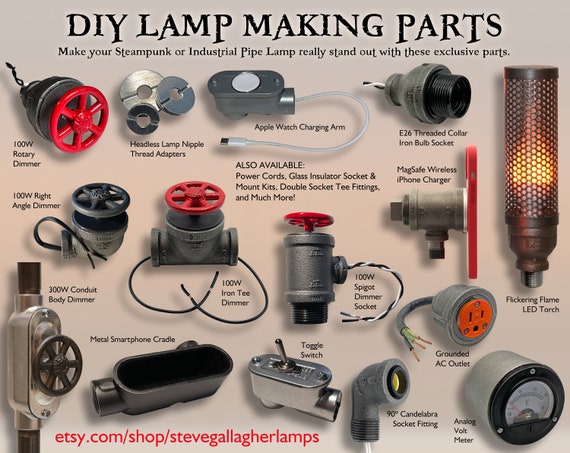This image showcases an extensive collection of DIY lamp-making parts designed to create standout steampunk or industrial pipe lamps. Highlighting the intricacy and variety of materials, it features numerous metallic mechanical components meticulously arranged with text descriptions beneath each part. Key elements include rotary dimmers with distinctive red valves connected to gray pipes, and a flickering flame LED torch designed to mimic a real flame. Among the unique fittings are headless lamp nipple thread adapters, Apple Watch charging arms, E26 thread collars, iron bulb sockets, and candelabra socket fittings with various wire connections. Detailed parts like right-angle dimmers, spigot dimmer sockets, and a 300-watt conduit body dimmer also make an appearance, along with a grounded red AC outlet surrounded by a bundle of wires. Additional notable items include an analog voltmeter, chrome toggle switches, and a metal smartphone cradle. At the bottom of the image, there is a link directing viewers to the Etsy website for purchasing these exclusive parts.